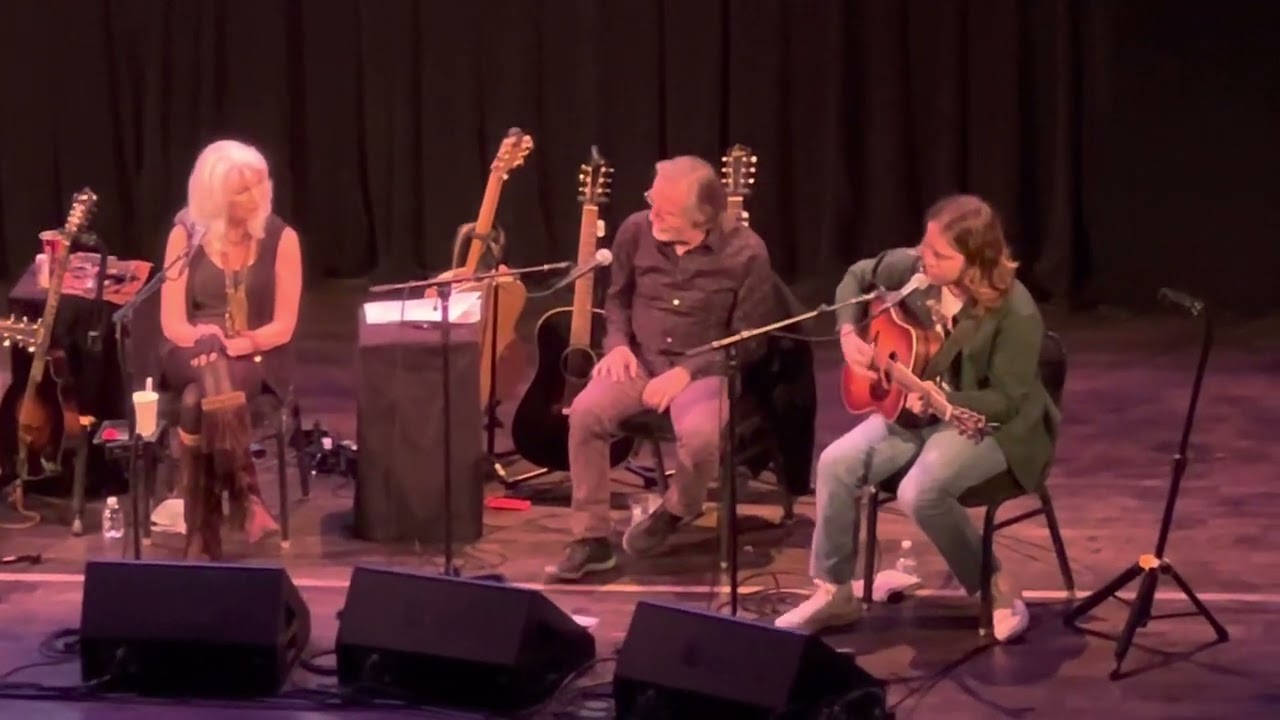The photograph captures an indoor musical performance, featuring three musicians on a modest grayish stage, illuminated by artificial light. The horizontally-oriented, full-color image reveals a backdrop of black curtains across the top, and three black speakers positioned at the front edge of the frame. Center stage sits an elderly white man with gray hair and glasses, dressed in a black button-up shirt, brown pants, and black shoes. He is slightly slouched and looks towards the woman on the left. 

To his left is an older white woman with white-gray hair, dressed in a black tank top or dress, and wearing fingerless gloves and leather boots. She sits with her hands in her lap, legs crossed, and looks to the right, towards the man in the center.

To the right of the man is a younger woman with long hair parted in the center. She is clad in a green blazer over a cream-colored undershirt, and strums on an orange or light brown acoustic guitar, its dark green strap visible across her shoulder. Positioned in front of her face is a microphone, suggesting she is singing.

The stage is cluttered with musical equipment, including additional guitars on stands and various microphone stands directed towards the man and the woman on the left. The floor appears to be wooden with a purple tint. The multitude of wires strewn across the stage adds to the sense of an unplugged, casual performance where music is interwoven with conversation, indicating a blend of musical and spoken interaction among the performers.